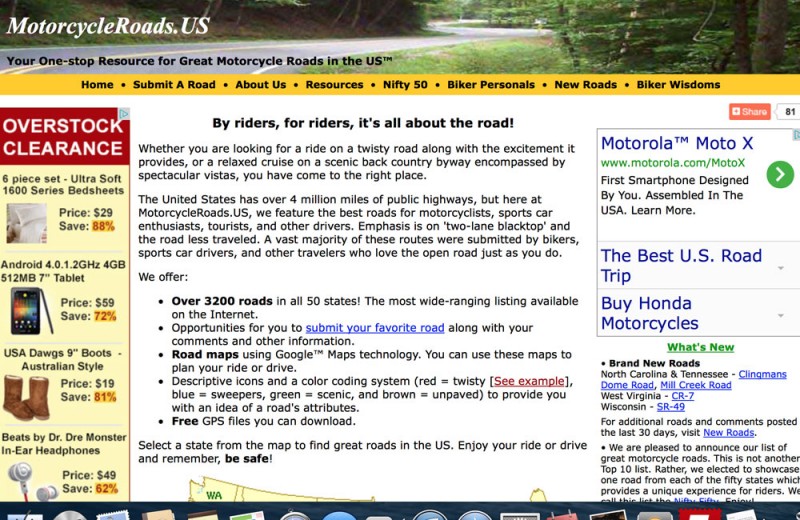Here is the cleaned-up and detailed caption:

---

The image showcases the homepage of the website MotorcycleRoads.us, designed as a comprehensive guide for motorcycle enthusiasts seeking the best roads in the U.S. At the top, a scenic photograph captures a winding road through a lush forest, setting an adventurous tone. 

Immediately below the website name, "MotorcycleRoads.us," displayed in bold black and white, is the tagline: "Your one-stop resource for great motorcycle roads in the U.S." A prominent yellow navigation bar with black text offers links labeled, from left to right: Home, Submit a Road, About Us, Resources, Nifty Fifty, Biker Personals, New Roads, and Biker Wisdoms.

On the left side of the page, an advertisement for Overstock Clearance showcases various items including a six-piece Ultrasoft 1600 Series bedsheet set, a 7-inch Android tablet, U.S. 8 Dogs 9-inch Australian-style boots, and Beats by Dr. Dre Monster in-ear headphones.

In the center, an inviting message in white text on a black background headlines with, "By Riders for Riders. It's all about the road." The text explains that whether one is looking for the thrill of twisty roads or a leisurely cruise through scenic byways with stunning vistas, MotorcycleRoads.us is the perfect destination. The site highlights the best routes from over 4 million miles of U.S. public highways, particularly focusing on two-lane blacktop roads and less-traveled routes. Descriptions and submissions are predominantly contributed by fellow bikers, sports car drivers, and other road enthusiasts.

Below the main text, a section titled "We Offer" includes bullet-pointed services provided by the site. To the right side of the content area, additional advertisements served by Google are visible, adding to the site's commercial elements.

---

This caption provides a detailed yet concise description of the elements within the image, giving readers a clear sense of the website's focus, design, and features.